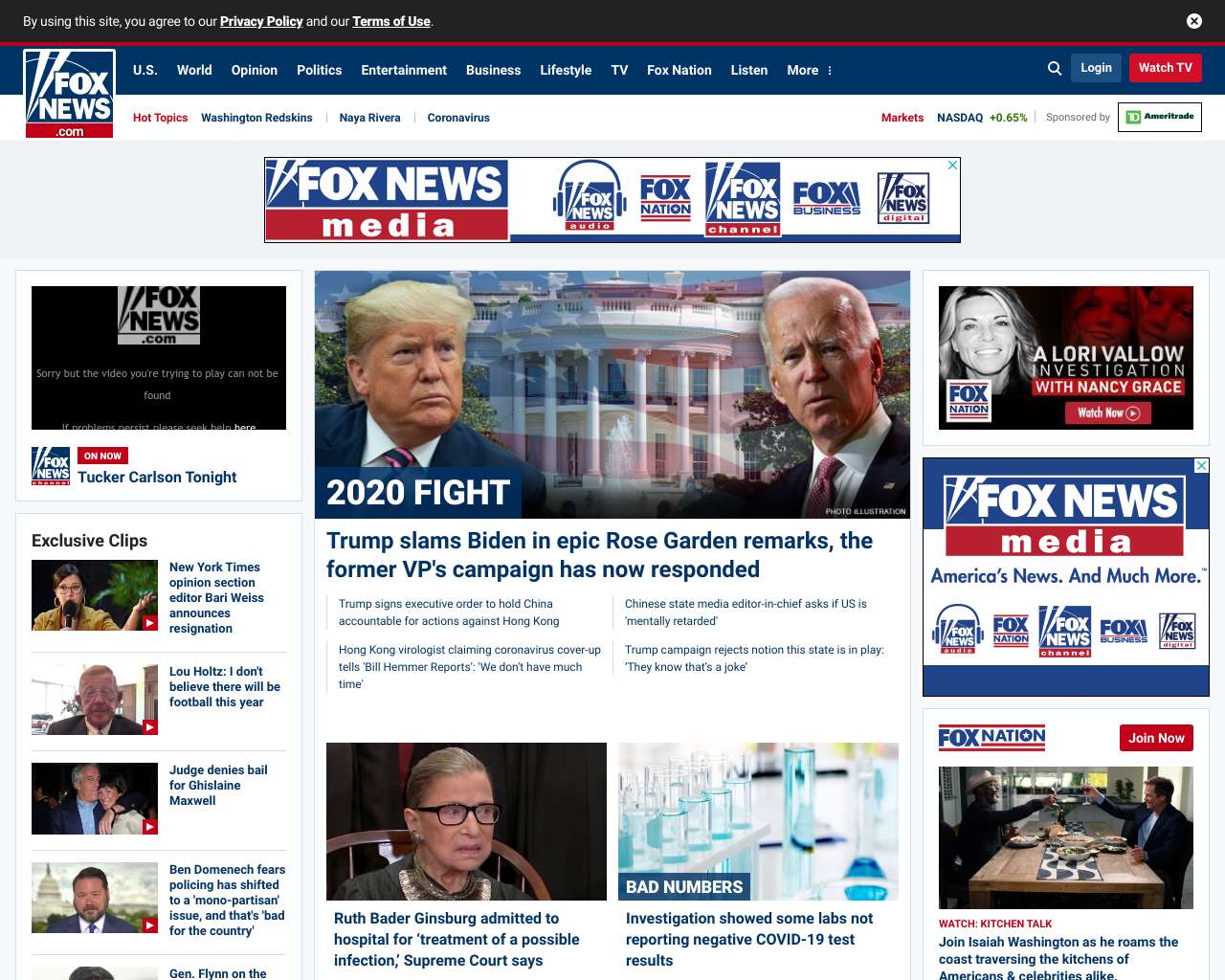This is an image taken from the Fox News website. At the top of the image, the iconic Fox News logo is displayed, featuring a two-tone design with a blue upper half and a red lower half. The text "Fox News" is emblazoned in white within the logo. Directly above this is a black border containing a privacy policy link. Below the logo, a red stripe is followed by a blue stripe, which includes a login option and a prominent "Watch TV" button highlighted in a red box.

Beneath these elements lies the Fox News Media banner, which showcases various Fox logos. Centrally positioned in the next segment is an image branded "2020 Fight," featuring pictures of Joe Biden and Donald Trump overlaying a semi-transparent image of the White House with an American flag. Below this, a headline reads, "Trump slams Biden epic Rose Garden remarks. The former VP's campaign has now responded."

On the left side of the image, a section indicates that viewers can currently watch "Tucker Carlson Tonight," listing the program's schedule. This area also offers exclusive clips for immediate viewing, with four visible video thumbnails and a fifth partially cut off.

The right side of the image features information about a Lori Vallow investigation, alongside an ad promoting Fox News Media, which describes it as "America's News and much more." Below this section, there's an advertisement for Fox Nation with an invitation to join the service. Further down, a headline notes that Ruth Bader Ginsburg has been hospitalized, followed by another story about an investigation into labs reporting negative COVID-19 test results.